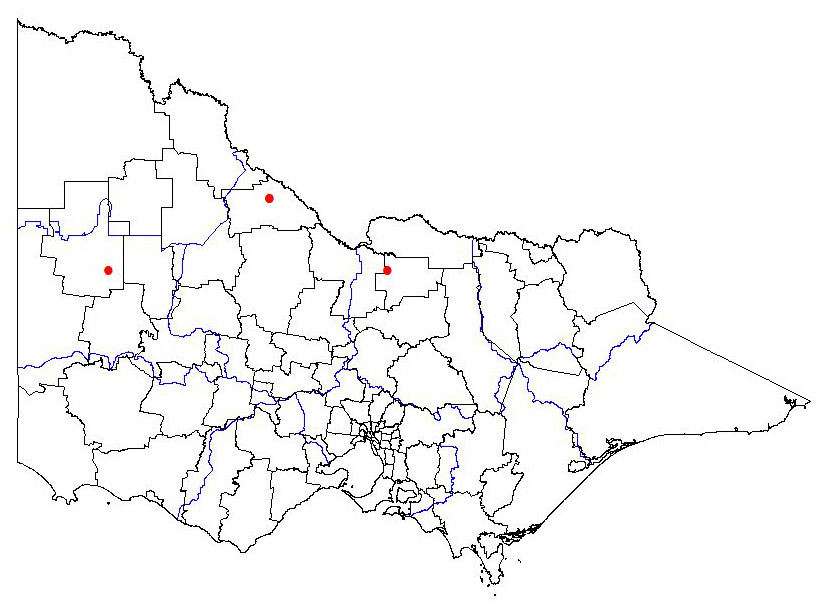The image depicts a map outlined with a black oblong, abstract shape resembling the end of a boot curving around. Inside this irregular exterior are numerous jagged black lines delineating various regions, which could be towns or districts. Additionally, blue lines are interspersed throughout, suggesting the presence of rivers or streams. Positioned within the map are three red dots, serving as markers or indicators. One red dot is located towards the left side, another near the top, and the third dot resides in the middle-right area. The map itself lacks explicit geographical identifiers, making it unclear which specific area it represents.